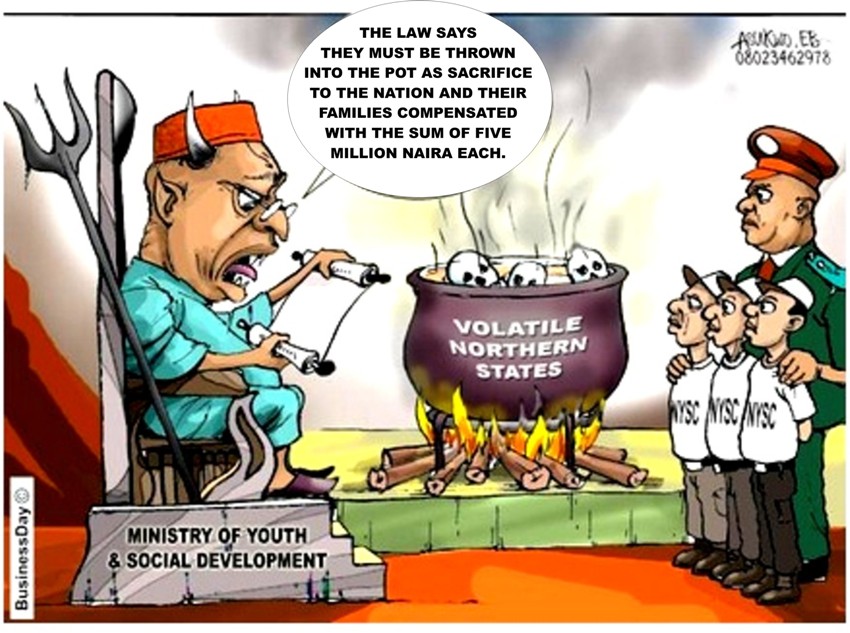The political cartoon is a wide rectangular image depicting a striking scene. On the left side, there is a man with brown skin, horns, a red cap, and a large head, seated on a gray throne labeled "Ministry of Youth and Social Development." He is clad in a blue robe and black slippers, holding a white scroll and speaking with an intense expression. A speech bubble from his mouth contains the ominous words: "The law says they must be thrown into the pot as sacrifice to the nation and their families, compensated with the sum of five million naira each."

In the center of the image is a large cauldron, labeled "volatile northern states," with wood and fire underneath and skulls popping out of it, symbolizing a dire and sacrificial process. 

To the right, a man with light brown skin in a green general's outfit stands with his arms on the shoulders of three smaller men, directing their attention towards the sinister figure on the throne. These smaller men are outfitted in white t-shirts emblazoned with "NYSC," and they wear caps with white tops and black brims.

Additional elements include text at the bottom left that reads "business day copyright," and handwritten text or a signature in the top right corner, adding to the official and editorial nature of the cartoon.